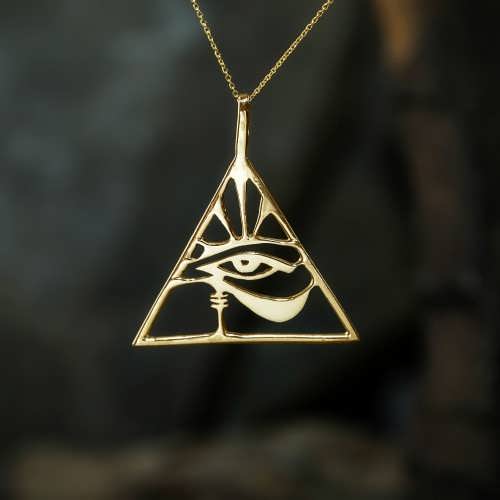The photograph depicts a square-shaped image focused on a gold necklace, featuring a pendant in the shape of a triangle. The pendant contains a detailed depiction of an Egyptian eye, also known as the Eye of Horus, with intricate designs including a swirl underneath moving leftward and lines resembling eyelashes extending from the top. The eye design within the triangular frame is meticulously soldered or welded, showcasing the skillful craftsmanship of a goldsmith. The pendant is suspended from a delicate, thin gold chain, hanging down centrally in the photograph. The background, appearing gray and black, is out of focus but features varying shades suggesting depth, and does not distract from the necklace which is the focal point. There are no gemstones on the pendant; it displays a simple, yet elegant flat yellow gold finish.